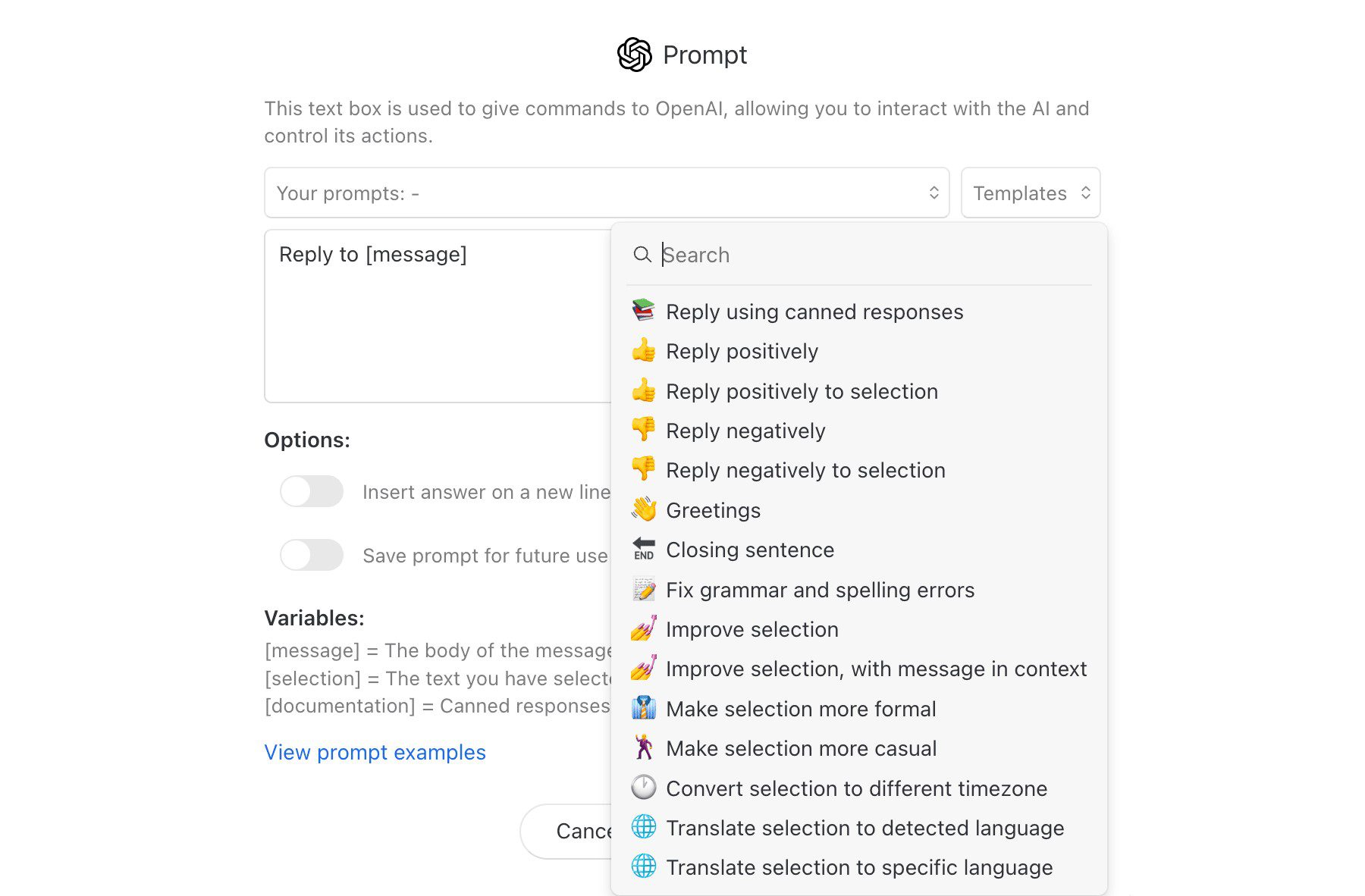This image showcases a user interface on a white background adorned with black text. At the top center, the word "Prompt" is displayed, accompanied by an icon resembling a flower. Below this title, a description reads, "This text box is used to give comments to OpenAI, allowing you to interact with the AI and control its actions." 

Beneath the description, there is a labeled section called "Your Prompts" and, to the right of this, a "Templates" box. Under the "Your Prompts" section, a white text box appears with the placeholder text, "Reply to message."

Further to the right, a search bar is located with various quick-action options listed underneath it. These options include: "Reply using canned responses," "Reply positively," "Reply positively to selection," "Reply negatively," "Reply negatively to selection," "Greetings," "Closing sentence," "Fix grammar and spelling errors," "Improve selection," "Improve selection with message in context," "Make selection more formal," "Make selection more casual," "Convert selection to different time zone," "Translate selection to detected language," and "Translate selection to specific language." Each option is accompanied by its respective icon to the left.

Below the "Reply to message" box, there are two additional options, both currently toggled off. The first option reads, "Insert answer on a new line," and the second says, "Save prompt for future use."